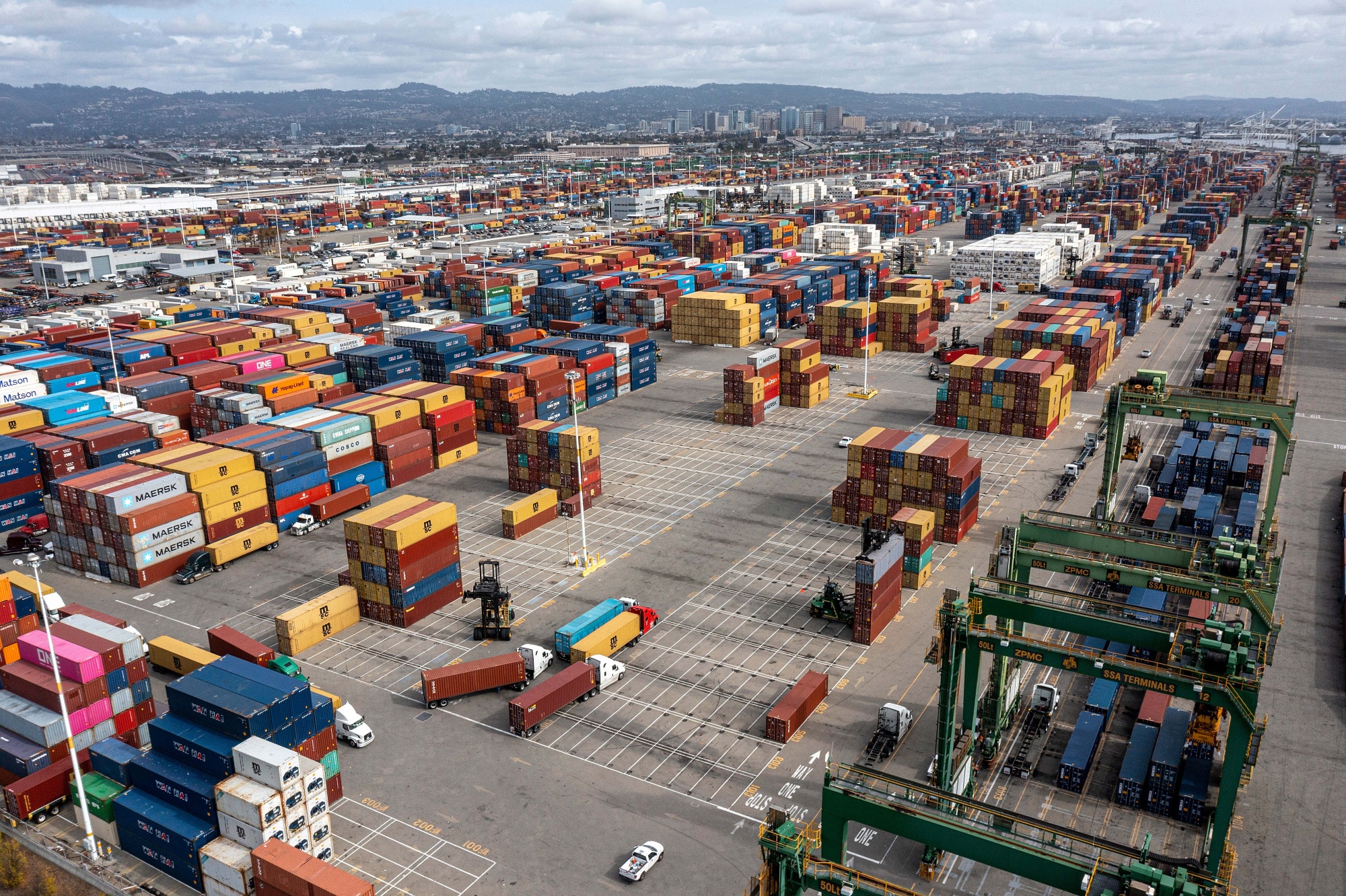The image depicts a sprawling, industrial cargo port captured from an overhead, top-down perspective. The vast asphalt surface is filled with rows upon rows of colorful shipping containers stacked four or five high, creating a vibrant mosaic. Towering cranes, including a giant green one, stand ready to load and unload these containers, emphasizing the area's bustling activity. Trucks are parked in designated areas, ready to transport their loads, but no people are visible within the shot. In the background, a cityscape with skyscrapers and hills can be seen under a clear sky, suggesting it’s a port city. The scene is illuminated by daylight, further highlighting the intricate details of this massive logistical hub.